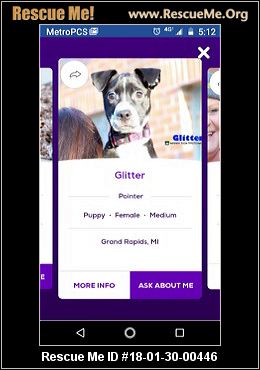In the image, Topless is in the foreground, engaged in rescuing activities as mentioned on the website www.rescuing.org. Charles is visible in the background, distracted by his phone displaying indicators such as Metro PCS, a clock showing 4G signal strength, a half battery icon, and symbols like "512," "X," and a "share" button.

A dog, with black fur and wearing a collar labeled 'Glitter,' is prominently featured. The top right of the image has 'Glitter' labeled, and below it, in purple text, it reads 'Pointer.' A line divides this section from the middle where it says 'Puppy, Female, Medium, Grand Rapids, Michigan' in white text. Additionally, there's an area highlighting 'Ask About Me,' with symbols for a left turn, a circle, and a square. Lastly, there is a Texas ID number '1801-300-446' next to the prompt 'Rescue Me.'